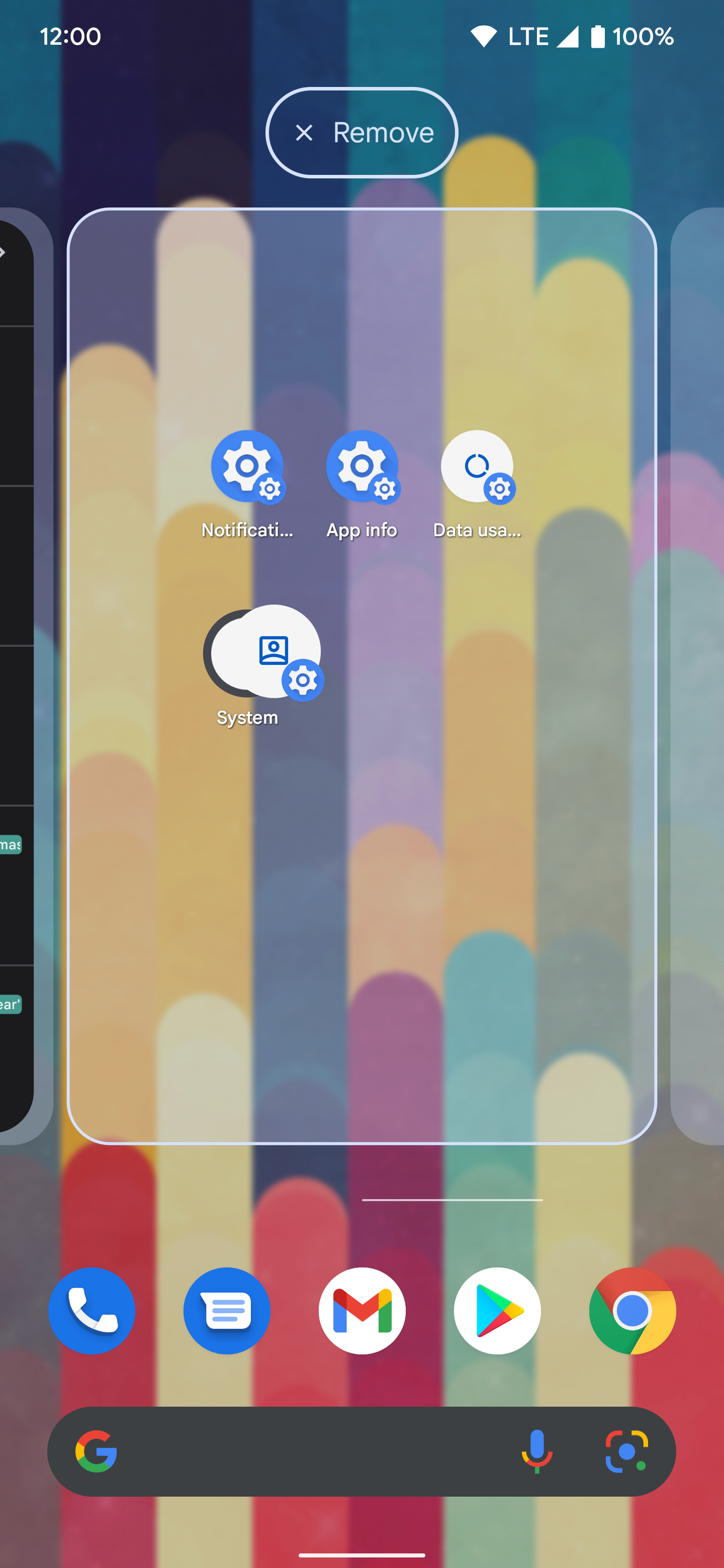The image is a screenshot of a smartphone's homepage. The background features an intriguing pattern of vertical stripes resembling cylindrical shapes, with each stripe composed of vibrant colors such as maroon, tan, and lavender. These colors are aesthetically arranged to create a visually appealing backdrop.

At the top of the screen, the current time is displayed on the left in white text, showing "12:00," though it is unclear whether it is noon or midnight. On the right, the battery indicator shows a full charge at 100%.

At the bottom of the screen, there is a dark gray Google search box with rounded corners. The multi-colored Google logo, represented by the letter "G," appears on the left side of the search box. Above the search box, several app icons are neatly lined up, including Phone and Messages (both with blue backgrounds), Gmail (white background), Google Play, and Google Chrome (a round icon with green, blue, yellow, and red colors).